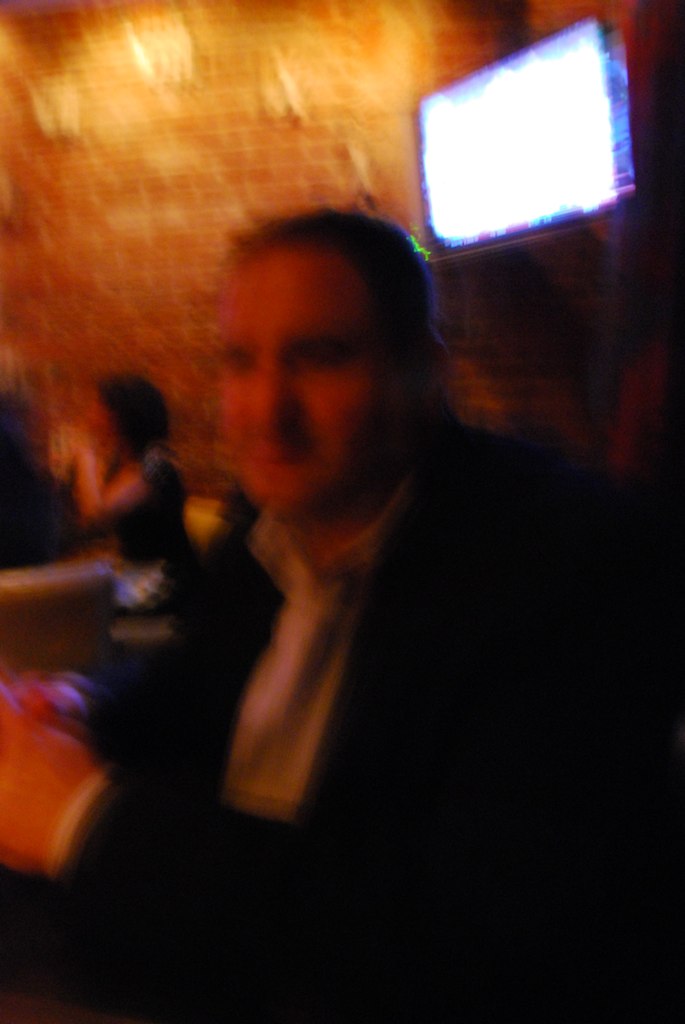In this blurry photograph captured in a restaurant or bar setting, a middle-aged man with a bald head is seated in the foreground. He is wearing a black blazer over a white undershirt. Behind him, a TV screen is mounted at the corner of an exposed red brick wall. In the background, a woman is seen sitting on a lounge chair with her hands over her face, seemingly engaged in conversation with someone. Due to the blurriness, the details of the man's face and other finer elements in the scene are indistinguishable.